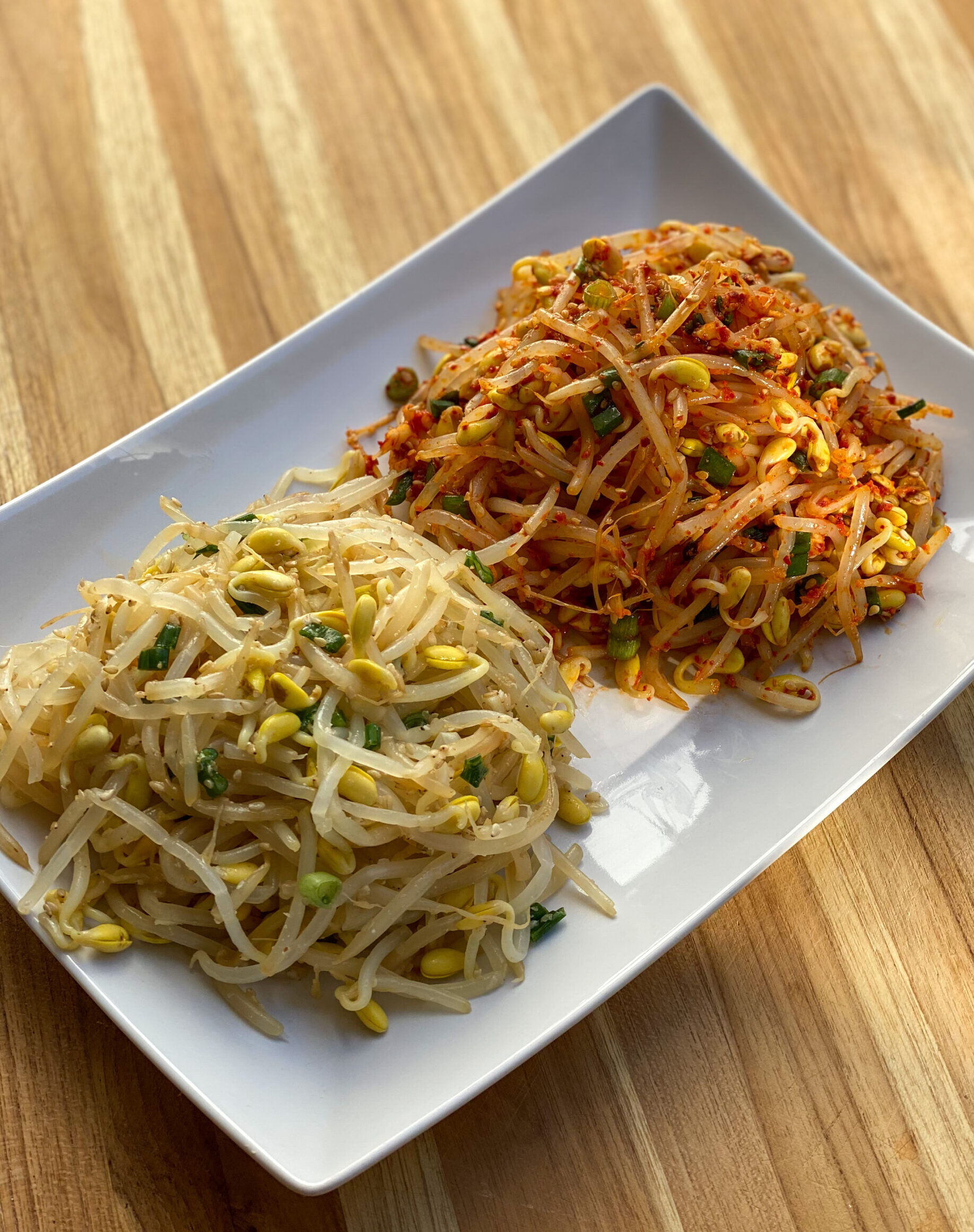The image depicts a white, rectangular plate with slightly curved edges placed on a light beige wooden surface, which has yellow streaks running through it. On the plate, arranged in mounds, are what appear to be spiced bean sprouts. The left side features yellow-colored sprouts, while the right side showcases sprouts with a red tint, indicating they're spiced and likely to be spicy. Small green flecks are scattered among the sprouts, adding to their visual appeal. The overall presentation suggests a carefully arranged and tasty-looking dish.